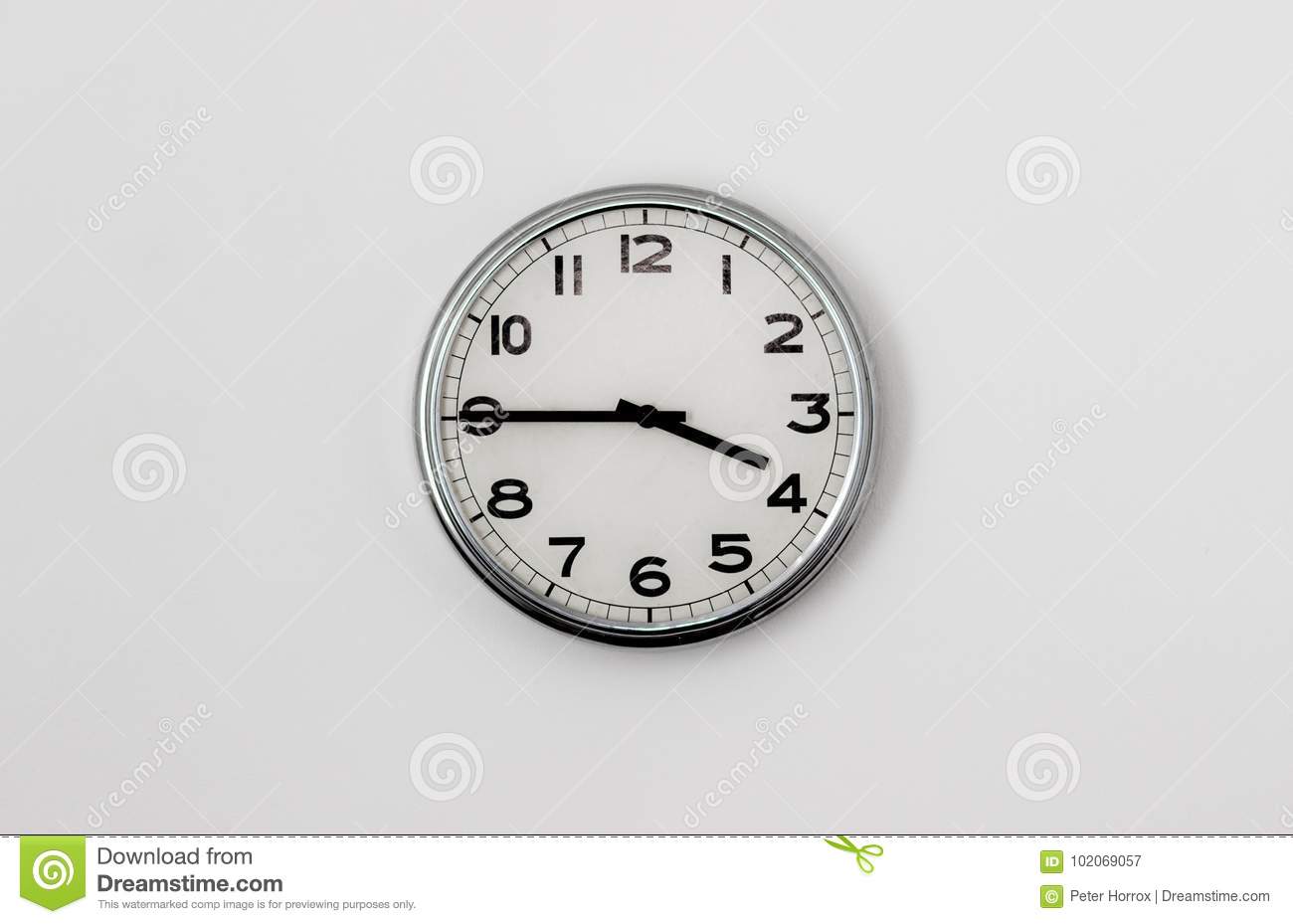The image showcases a round wall clock with a sleek silver frame. The clock's face is entirely white, featuring bold black Arabic numerals from 1 to 12, arranged in a traditional format with no Roman numerals. Overlaying the clock are several watermark designs, including six curly Q patterns and a grid of intersecting lines. The words "dreams time" are prominently displayed on the image, with additional text at the bottom reading "Download from dreamstime.com." There is also a toxic green-colored banner on the image, containing white font that states "ID" followed by a series of numbers. Additionally, a pair of green-handled scissors and a photo ID card appear in the design as well. Overall, this appears to be a watermarked stock photo, likely intended for advertising or digital use.